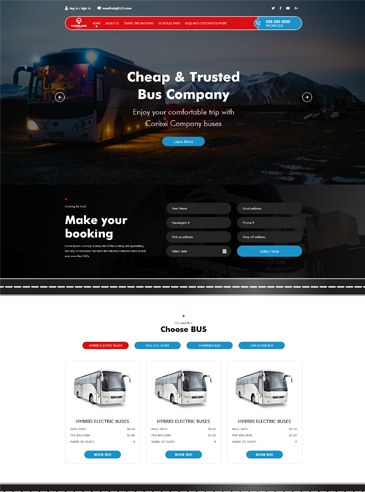Screenshot of the transportation website's homepage: The top half features a photograph of a large tour bus, positioned on the left side of the frame. The bus faces the camera and is slightly angled to the left, showcasing its vibrant blue lights at the top and an orange light at the bottom left, with additional darker orange lights along its side. Behind the bus, a picturesque ridge of blue, snow-capped mountains is visible. The image has a darkened overlay, with large white text that reads, "Cheap and Trusted Bus Company," followed by smaller white text saying, "Enjoy your comfortable trip with Connexi Company Buses." 

A blue button with blurry white text is positioned beneath this message. At the top of the image, there is a red header with rounded edges and a thin white outline, extending into a medium blue section on the right with white text. 

Below the photograph, a section on the left displays large white text that says, "Make Your Booking." To the right are eight medium gray, rounded-sided text entry boxes, filled with illegible blurry white text. The bottom right text box is distinctively blue, resembling a button, and features white text.

The lower portion of the page has a white background, presenting three selection screens, each displaying a picture of a different bus model.